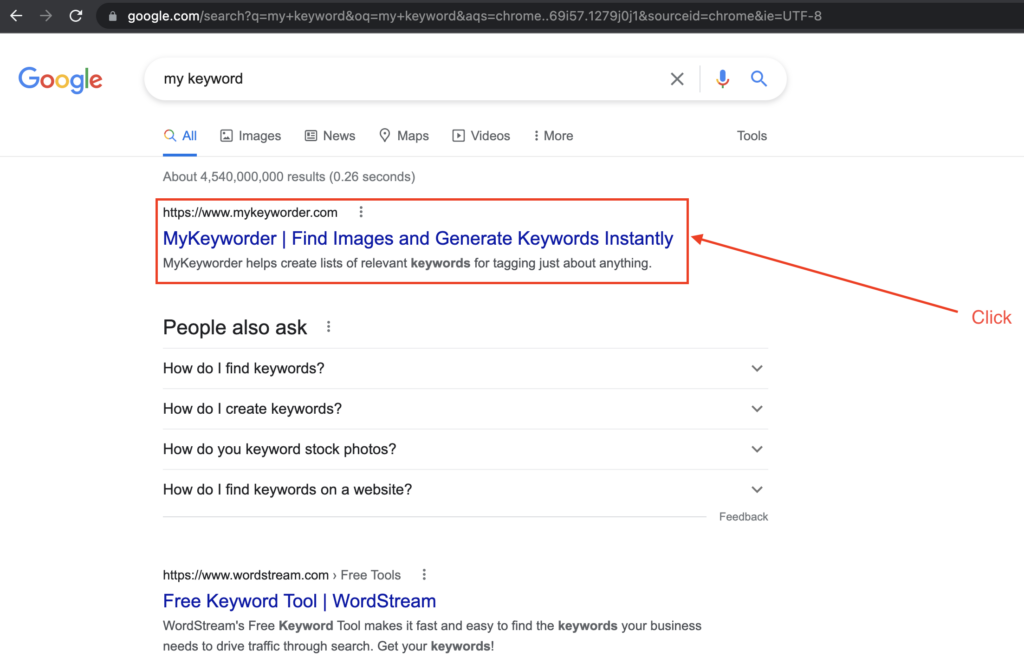This image is a detailed screenshot from the Google search engine results page, displaying a web browser with a black address bar featuring white text and the website URL. The remaining portion of the image showcases a webpage with a white background. 

In the top left corner, the iconic Google logo is present, showing in blue, red, yellow, and green sequentially. The user searched for the term "my keyword" which is visible within the search box at the top. Directly beneath the search box, the primary search result is from the website "www.mykeyworder.com." 

The headline reads "MyKeyWorder" (formatted as a single word) followed by the tagline "Find images and generate keywords instantly." Below this, a brief description in gray font states, "MyKeyWorder helps create lists of relevant keywords for tagging just about anything." This entire section has been emphasized by a red box drawn around it. Additionally, on the right side of the highlighted area, the word "click" is displayed with an arrow pointing directly to the box, suggesting further action.